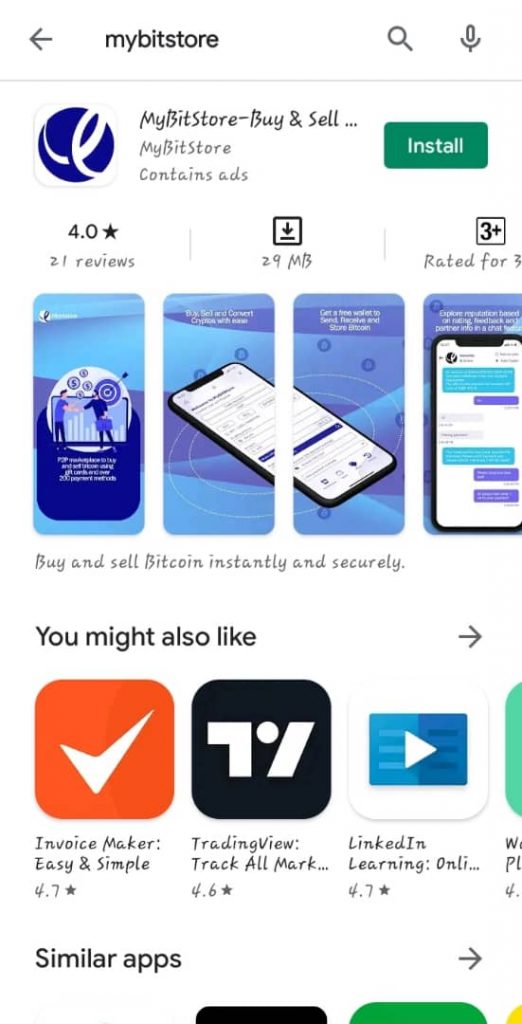Screenshot of a mobile app store page for "MyBitStore." At the top left, there's a back arrow icon. Along the top right, there are a magnifying glass and a microphone icon to facilitate voice search. Below, the app title "MyBitStore" appears in lowercase on the left, while on the right, there is a green "Install" button. The title "MyBitStore - Buy and Sell..." is displayed next to an app icon, followed by a notification that the app contains ads. The distinctive feature of this screenshot is the customized italicized font used throughout due to the user's phone settings.

Further down, app details such as reviews, file size, and ratings are mentioned, though somewhat cropped out on the right side. Centered in the screenshot are four thumbnail previews of the app's interface, each scaled to fit a mobile screen. Beneath the thumbnails, in bold text, it reads: "Buy and Sell Bitcoin Instantly and Securely," indicating the app's core purpose. At the bottom of the screenshot, a section titled "You Might Also Like" showcases thumbnail suggestions for other related apps.